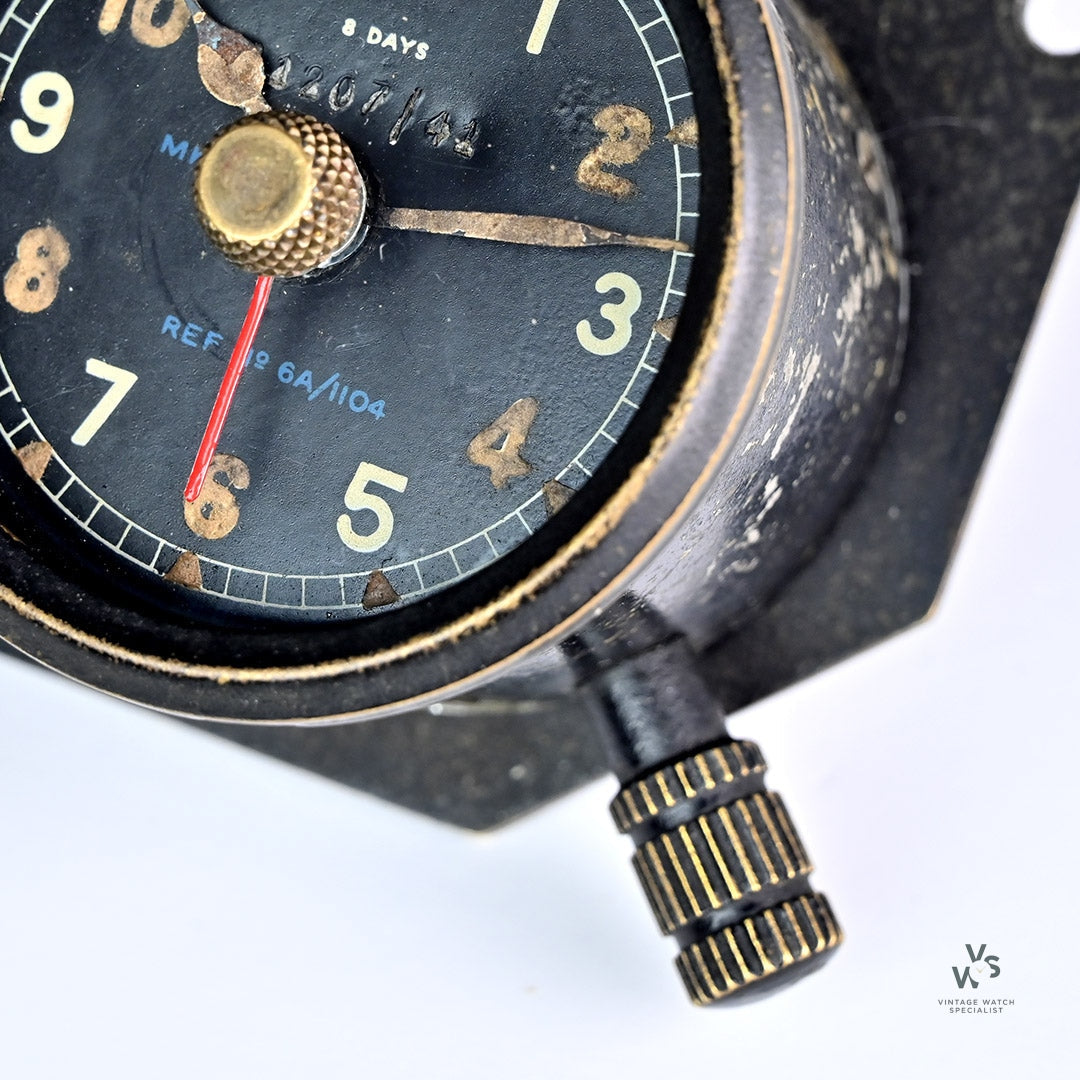The image depicts an aged watch face, characterized by its worn and faded features. The dial displays numbers from 1 to 10, with the number 2 notably faded, alongside worn text indicative of its prolonged use. The face is black with cream and brown numerals, and it bears the words "8 days" and "REF 6A/1104" in blue. The watch hands include a red second hand pointing towards the 6, a slim minute hand between the 2 and 3, and a shorter hour hand at the 10. A golden knob adjacent to the letters "MV" is also visible. The watch has a vintage aesthetic, exacerbated by the faded gold elements and chipped black coating. The overall condition of the watch hints at extensive wear and historical significance. The watch face is set within an octagonal background, resembling a gauge or tire pump with white and black ridged nozzles. The bottom right corner houses a logo related to vintage watch specifications.